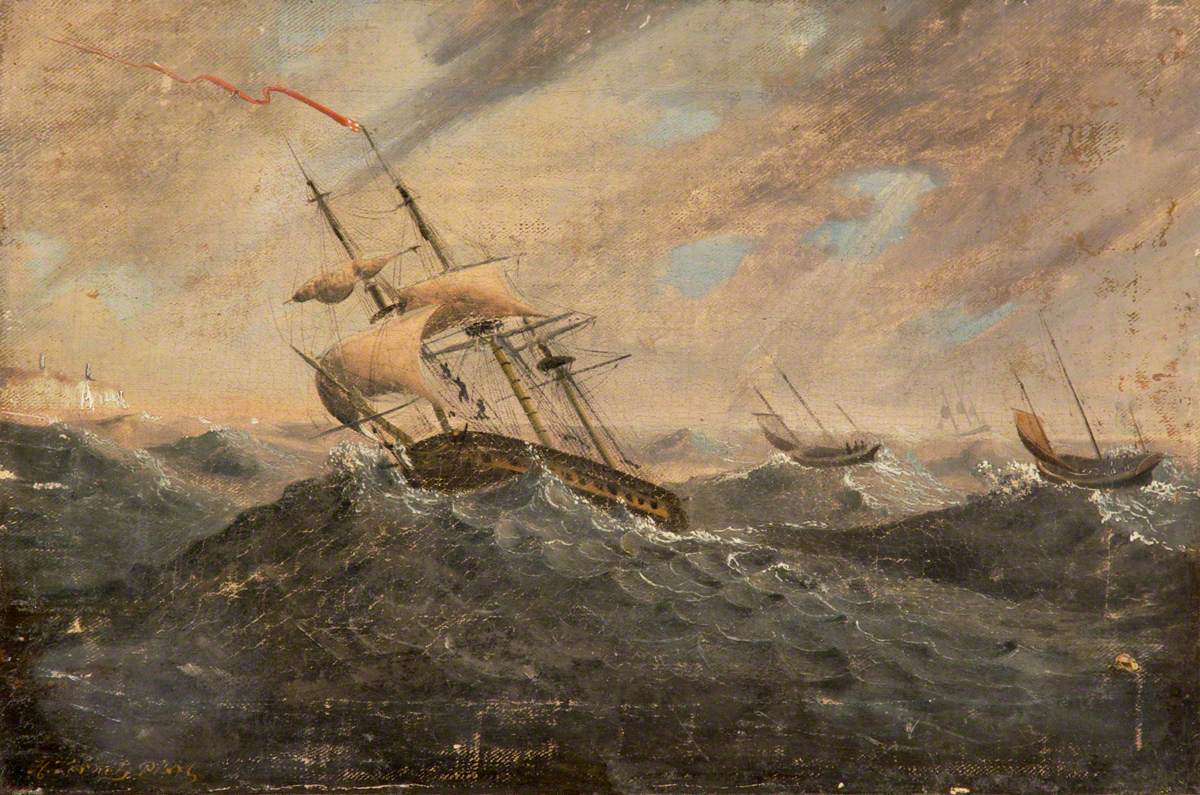This painting depicts a turbulent maritime scene, capturing several ships struggling against rough, choppy waters. The central focus is a large, brown vessel with its three sails dramatically furled and unfurled, cresting a monstrous wave. The ship is heavily tilted to the left, with a red banner trailing from one of its top masts. Deckhands are visible, clinging to the ropes amid the tumultuous conditions. Surrounding this main ship are at least three to four more vessels—some smaller, curved boats, each also tilted precariously. The waters are depicted in shades of gray and black, punctuated with white sea foam, reflecting the ferocious sea. On the right side of the image, something floats in the water, suggesting possible debris from one of the ships. The sky is predominantly dark and cloudy with streaks of brown and orange, hinting at a brewing storm, though patches of blue sky peek through. The background features the suggestion of land on the left, possibly illuminated by a distant ray of sunlight, adding a striking contrast to the otherwise dramatic scene.